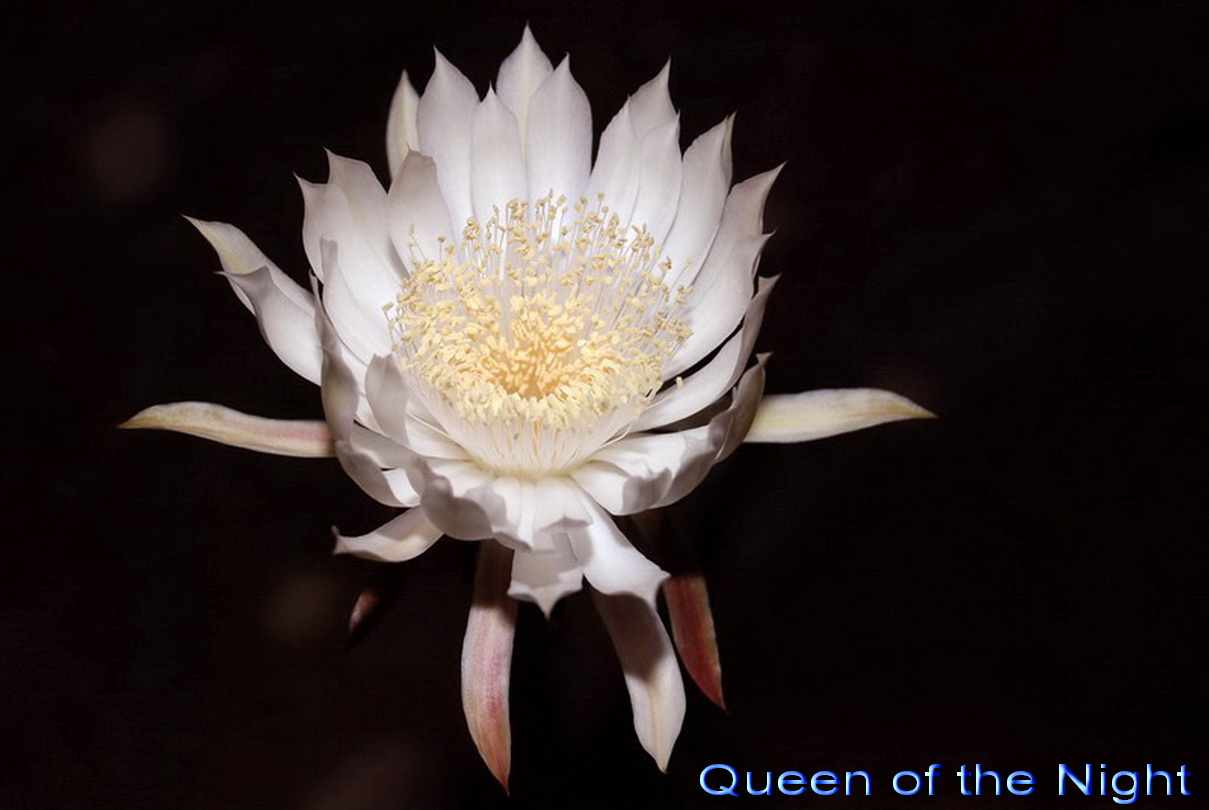This captivating photograph showcases a striking white flower, likely an orchid, in full bloom against a stark black background. The flower, referred to as the "Queen of the Night" in blue lettering on the lower right-hand corner, boasts over a dozen overlapping, off-white petals. Some of these petals are spread wide, creating an impression of open arms eagerly awaiting an embrace, while others swirl gracefully in various directions. At the heart of the blossom, slender stalks are visible, suggesting the presence of pollen where a bee might land. The high contrast between the delicate, intricate structure of the flower and the dark backdrop makes this image particularly artistic and visually arresting.